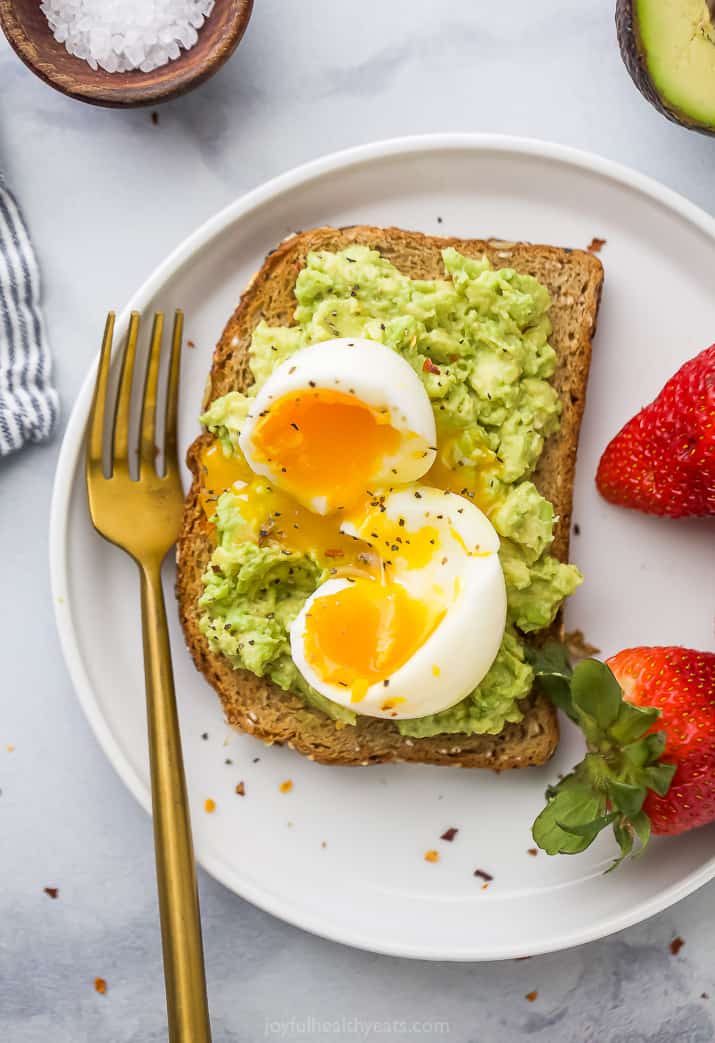In the image, a round white plate with a thin, slightly elevated rim and a modestly deeper center is prominently displayed, occupying approximately 80% of the frame with a portion on the right side cut off. Centered on the plate is a piece of toasted bread generously spread with chunky avocado. Atop the avocado sits a soft-boiled egg, split open to reveal its runny yolk, which is oozing out enticingly and dusted with a sprinkle of pepper for added flavor. Flanking the toast on the right side are two vibrant red strawberries. Meanwhile, to the left of the plate, a metallic fork with a long handle lies elegantly.